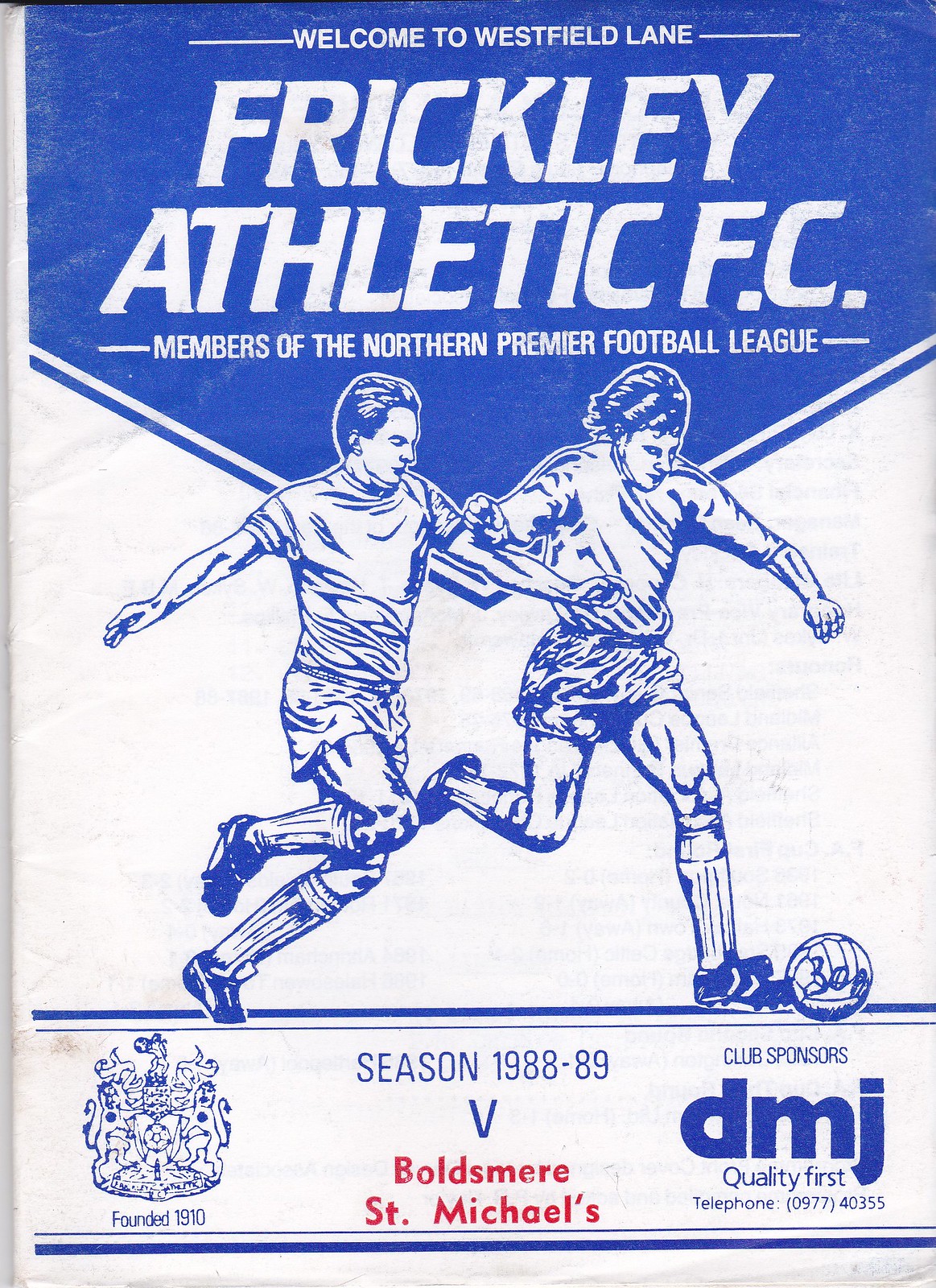This image appears to be a detailed poster for a football club, specifically a program cover for a soccer game. Dominated by blue and white colors, it prominently features the text "Welcome to Westfield Lane" at the top. Large text underneath reads "Frickley Athletic FC," and smaller text declares the club's membership in the Northern Premier Football League. A central illustration depicts two football players in action, vying for a ball. The bottom text indicates the match details: "Season 1988-89, versus Boldsmere St. Michael's," with "Boldsmere St. Michael's" highlighted in red at the center bottom. The left side features a crest adorned with two lions and a soccer ball, indicating the club's founding year of 1910. On the right, sponsorship information is listed: "Club Sponsors: DMG Quality First, Telephone 0977 40355."